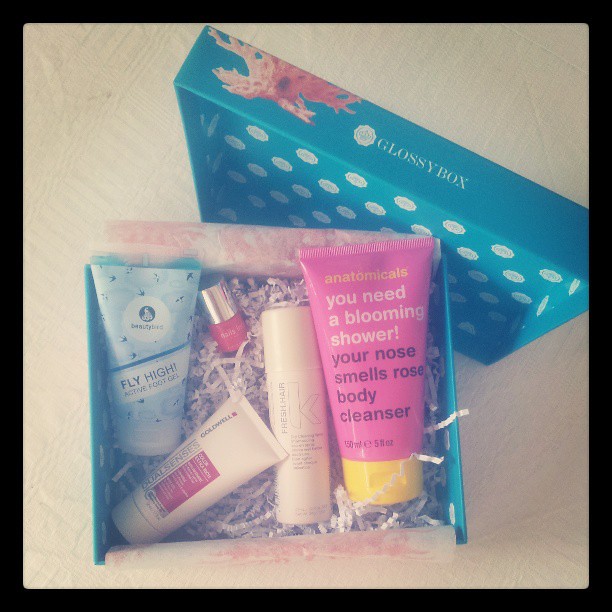The image is a top-down photograph of an open aqua blue box with the lid tilted against the base. The interior lid of the box has white polka dots, and the lid features "Glossy Box" written in the center. The box is filled with various beauty care items nestled on a bed of shredded newspaper, likely for cushioning during shipping. 

Starting from the left, there is a light blue squeeze tube labeled "Fly High Active Foot Gel" in dark blue font with a white circle at the top, which appears to say "Beauty Bed," though the text is small. Below it is a white bottle labeled "Dual Sensors Goldwell," with additional text that's too small to read, placed on a red rectangle background.

To the right of these items, there's a red bottle with a gold cap, which might be a nail polish. Adjacent to it is a small cream-colored spray bottle with black text, again too small to decipher. In the center, there's another white cylindrical item, labeled "Fresh Hair" with a prominent "K."

On the right, there's a pink squeeze tube labeled in yellow as "Anatomicals" and reads "You Need a Blooming Shower!" followed by "Your Nose Smells Rose Body Cleanser" in black text. The tube has additional labeling indicating "five floral ounces" and features a yellow circular cap at the bottom.

Surrounding these items is shredded paper to keep them in place, and the box sits on a cream-colored surface. The photo is bordered with a black edge.